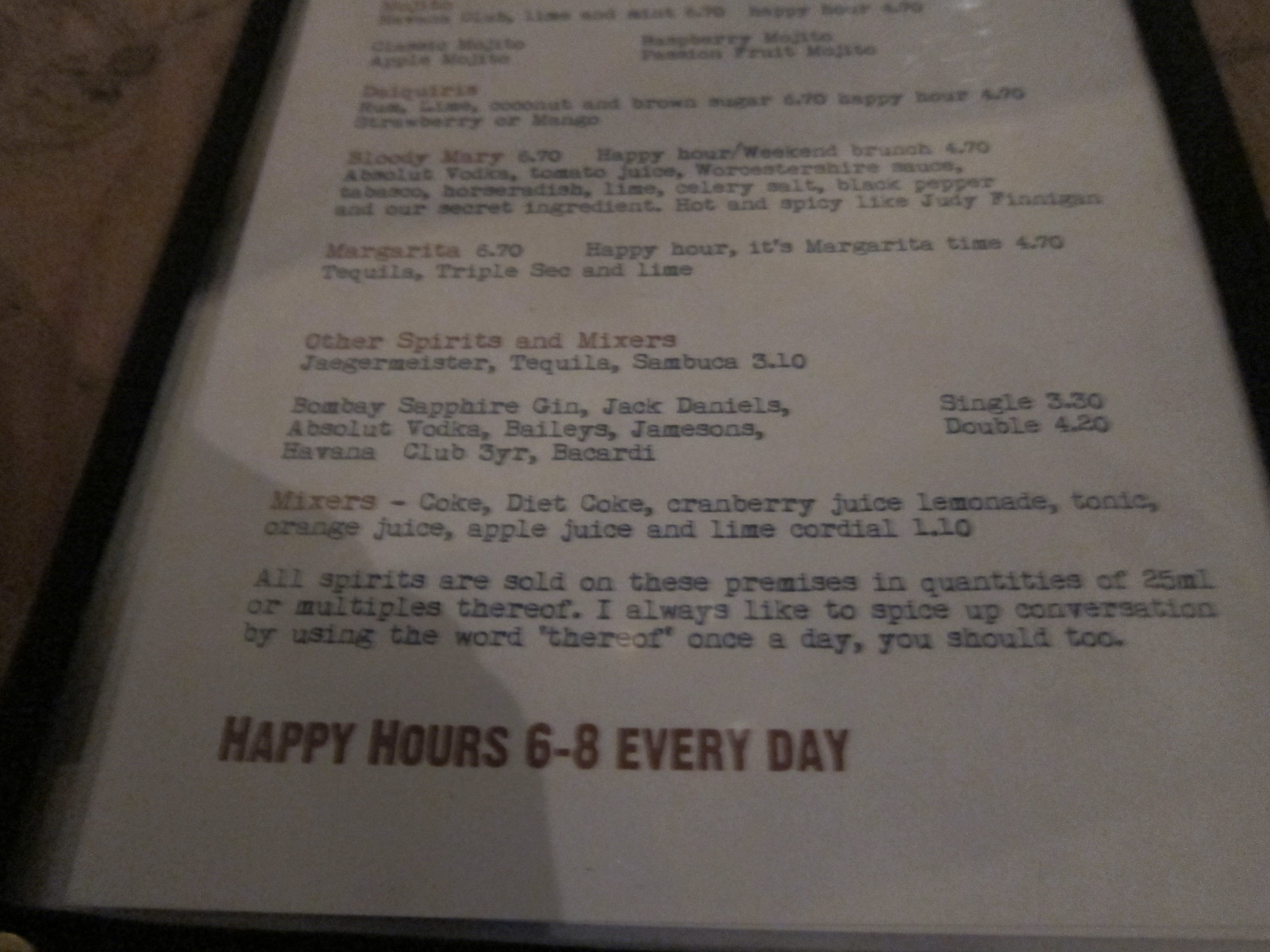This color photograph captures a drink menu from an unidentified bar. The image shows a white menu with a black border, featuring blue font for the text and red outlines highlighting the drink options. There is a noticeable shadow in the bottom left corner. The menu includes various typical cocktails such as daiquiris, Bloody Marys, and margaritas, along with an assortment of spirits and mixers like Bombay Sapphire Gin and Jack Daniels, each priced at $3.30. Specific details such as a margarita priced at $6.70, and a happy hour margarita at $4.70, indicate both regular and discounted prices. At the bottom of the menu, emphasized in red text, is the happy hour timing: "6-8 every day." Additionally, the menu notes that all spirits are sold in quantities of 25ml or multiples thereof.